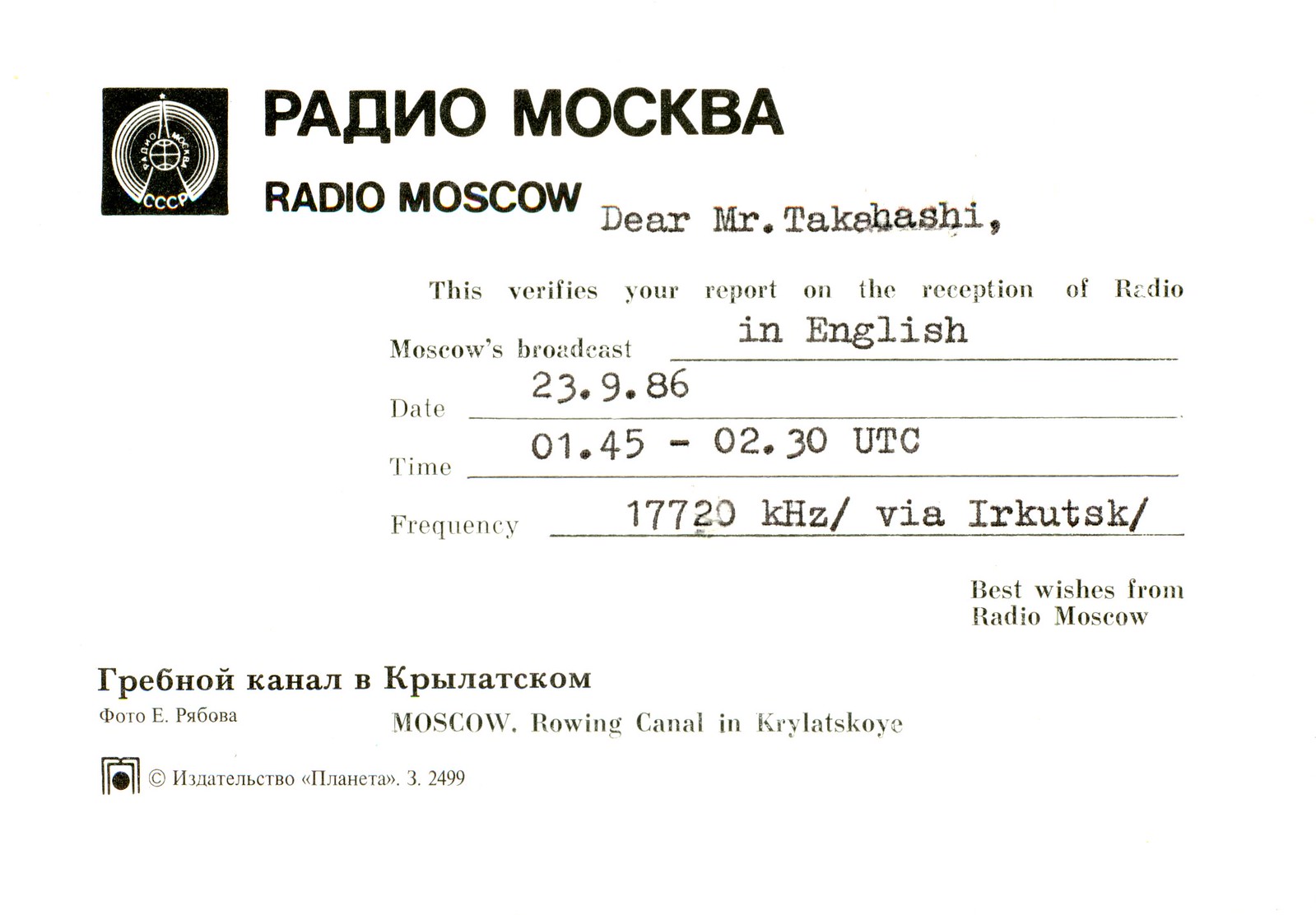A detailed memo or note appears to be an acknowledgment of a radio program reception. In the top right-hand corner, there is a logo with the letters "CCCP" and accompanying Russian text. Below this, it says "Radio Moscow." The document begins with "Dear Mr. Takahashi," and it verifies the receipt of a report on the reception of Radio Moscow's broadcast in English. The broadcast details are as follows: date 23-9-86, time 01.45 to 02.30 UTC, and frequency 17720 kHz via ERC stick. The note extends "Best wishes from Radio Moscow." At the bottom right-hand corner, there is another portion of Russian text and a second logo with a copyright symbol. The words "Moscow, Rowing Canal, and Krylatskoye" are printed in English. The document has black lettering against a white background, with certain elements typed in dark letters.